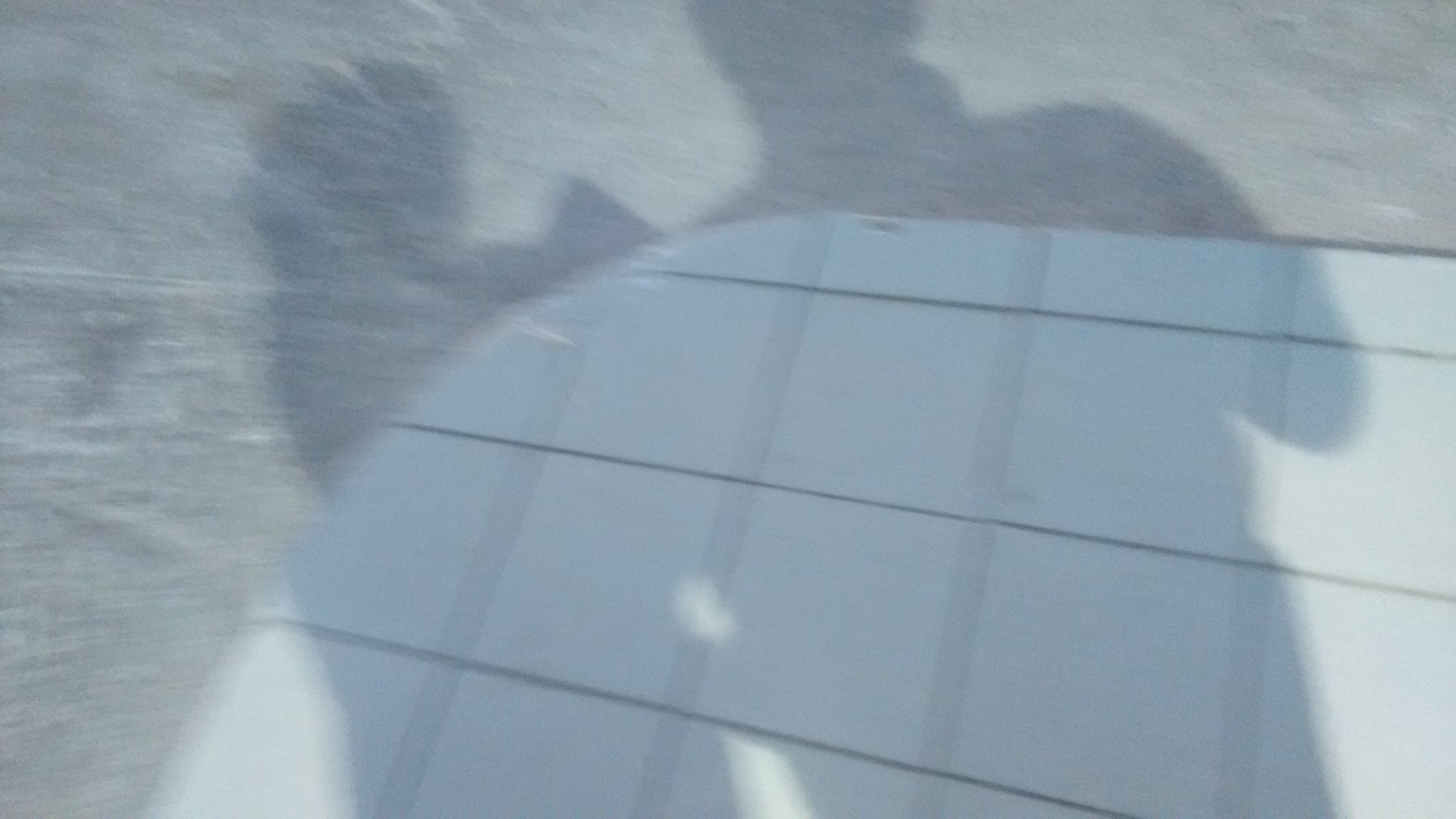The photograph captures a downward perspective of a floor transitioning from a white tiled section to a gray concrete area. The white tiles are full squares except for the last row at the top, which features half-width tiles, and the side row, which has three-quarter-width tiles. At the corner, the tiles curve, forming partial triangular shapes. The scene includes the shadows of two individuals; one on the right standing straight ahead, and the other on the left, slightly turned in a side profile. The contrast between the clean, geometrically-patterned tiles and the plain concrete creates a distinct visual separation between the two areas.